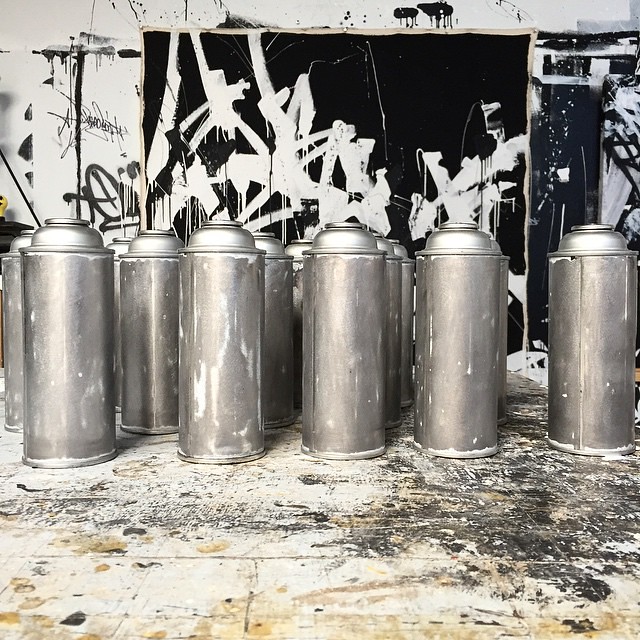The image is a color photograph depicting what appears to be an art studio in disarray. The floor, which is tiled, is heavily splattered with a chaotic mix of old, dried paint and ink in shades of black, orange, beige, and brown, lending it a heavily used, grimy appearance. Dominating the middle and stretching toward the background are numerous cylindrical metal containers, resembling old milk pails, each tapering into a bell shape at the top. These containers are arranged in rows, with five prominently visible in the forefront and additional ones arrayed behind them, totaling around fifteen. They are silver and appear to be well-used, possibly as containers for paint; their tops are missing, adding to their utilitarian look.

In the background, the setting hints at the chaos of artistic creation. Various surfaces, including what could be boards leaning against the back wall, are heavily splattered with paint and display spray-can graffiti, featuring black and white streaks and splashes. There is an uneven wooden border encircling a section of the canvas or board from the right top corner down to the left side, vanishing behind the tall silver containers, further framing the scene. The background wall is predominantly white, marred with sporadic blotches of paint as if someone has been experimenting with spray paint, enhancing the atmosphere of creative disorder. A prominent black canvas or board also stands out, marked by abstract white lines suggestive of graffiti, but without any distinct, legible words.